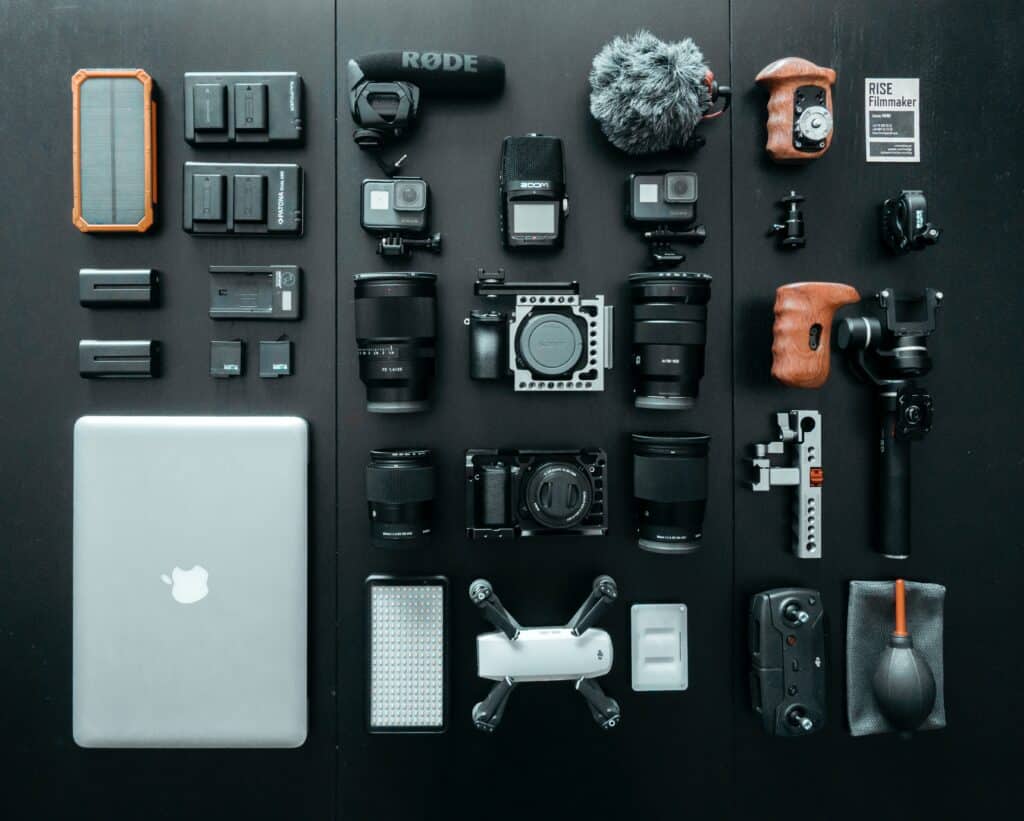This detailed color photograph showcases an impressive array of camera and filmmaking equipment meticulously arranged on a black surface composed of three connected panels. 

### Left Panel:
At the top, a rectangular wooden flash is prominently positioned, beside two battery chargers, each holding two batteries. Below these, additional batteries and a solo battery charger can be spotted. Further down resides an Apple MacBook in the bottom left corner, with two small memory card-like squares above it.

### Middle Panel:
Dominating the center panel, a hairy microphone cover and a microphone featuring a small screen are flanked by two GoPro cameras—one gray and black, the other all black. Between and surrounding these are two sets of camera lenses and another flash. An oval-shaped drone with four legs and a small, somewhat white rectangular object lie below the cameras. LED portable light systems fill out this section.

### Right Panel:
In the top right corner, a square item marked "RISE Filmmaker" leads the collection of wooden hand grips, black mics or connectors, and two tripods—one black, one gray. A black joystick controller is situated beneath these, while at the bottom right, a gray rag with a black and brown bulb meant for cleaning lenses joins the scene. Additionally, a portable solar charger battery backup unit and remote control for the drone underline the practical and comprehensive nature of this filmmaker’s toolkit.

All these professional tools and accessories are neatly organized, showcasing the readiness and versatility required for diverse filming activities.